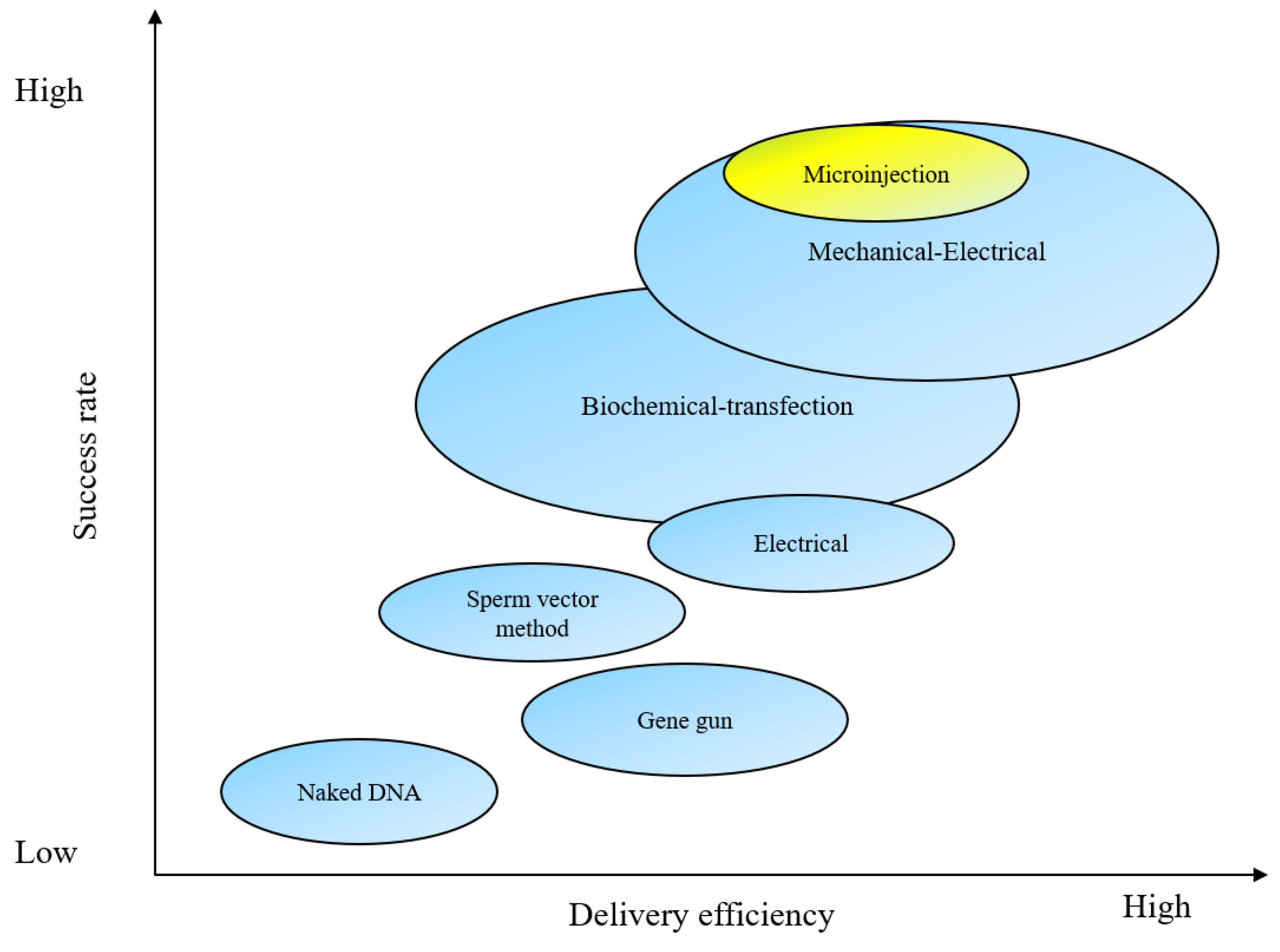This image is a detailed diagram depicting various methods of genetic material delivery, plotted on a graph with the x-axis labeled "Delivery Efficiency" and the y-axis labeled "Success Rate," both ranging from low to high. The diagram features a series of blue circles, except for one yellow circle, each labeled with a different delivery method. Starting from the bottom left and moving upward, the circles are labeled: Naked DNA, Sperm Vector Method, Gene Gun, Electrical, Biochemical Transfection, Mechanical-Electrical, and Microinjection. The background is white, emphasizing the visual representation of these methods' comparative efficiencies and success rates on a clear, uncomplicated backdrop. The placement of these labels suggests an assessment or comparison of various experimental fertilization or gene delivery techniques.